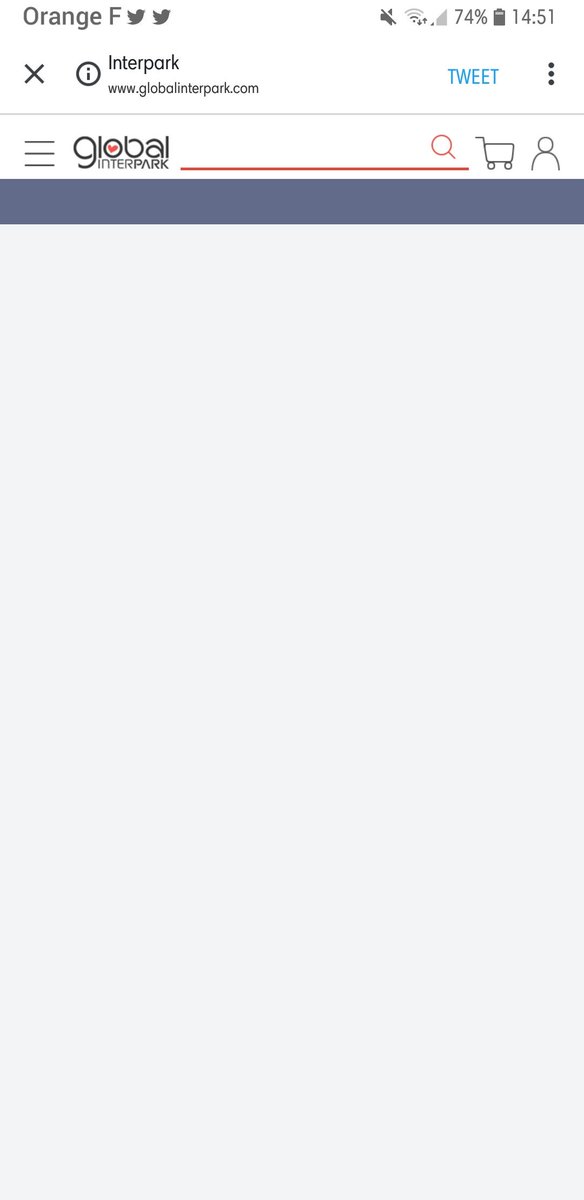This detailed caption describes an image that shows a screenshot of a cell phone displaying a web page. 

At the upper left corner of the screen, there is grey text that reads "Orange F," accompanied by two grey Twitter birds. In the upper right corner, notifications are turned off, and next to this, there are icons showing Wi-Fi strength, a battery icon indicating 74% charge, and the current time displayed as 14:51.

Below this top bar, on the left side, there is a grey "X" symbol. Adjacent to it, to the right, is the URL "Interpark," specifically www.globalinterpark.com, written in black text. On the same line, positioned to the far right and in blue text, is the word "Tweet."

Below this section, there is a light grey horizontal line separating it from the rest of the content. Directly beneath this line, we see the logo for "Global Interpark," which is intricately designed. The text "Global" has a small red heart inside the letter "O," adding a touch of detail to the design. To the right of the logo, there are icons for navigation: a red magnifying glass representing search, a black shopping cart for purchasing items, and a person icon presumably for user account or profile access.